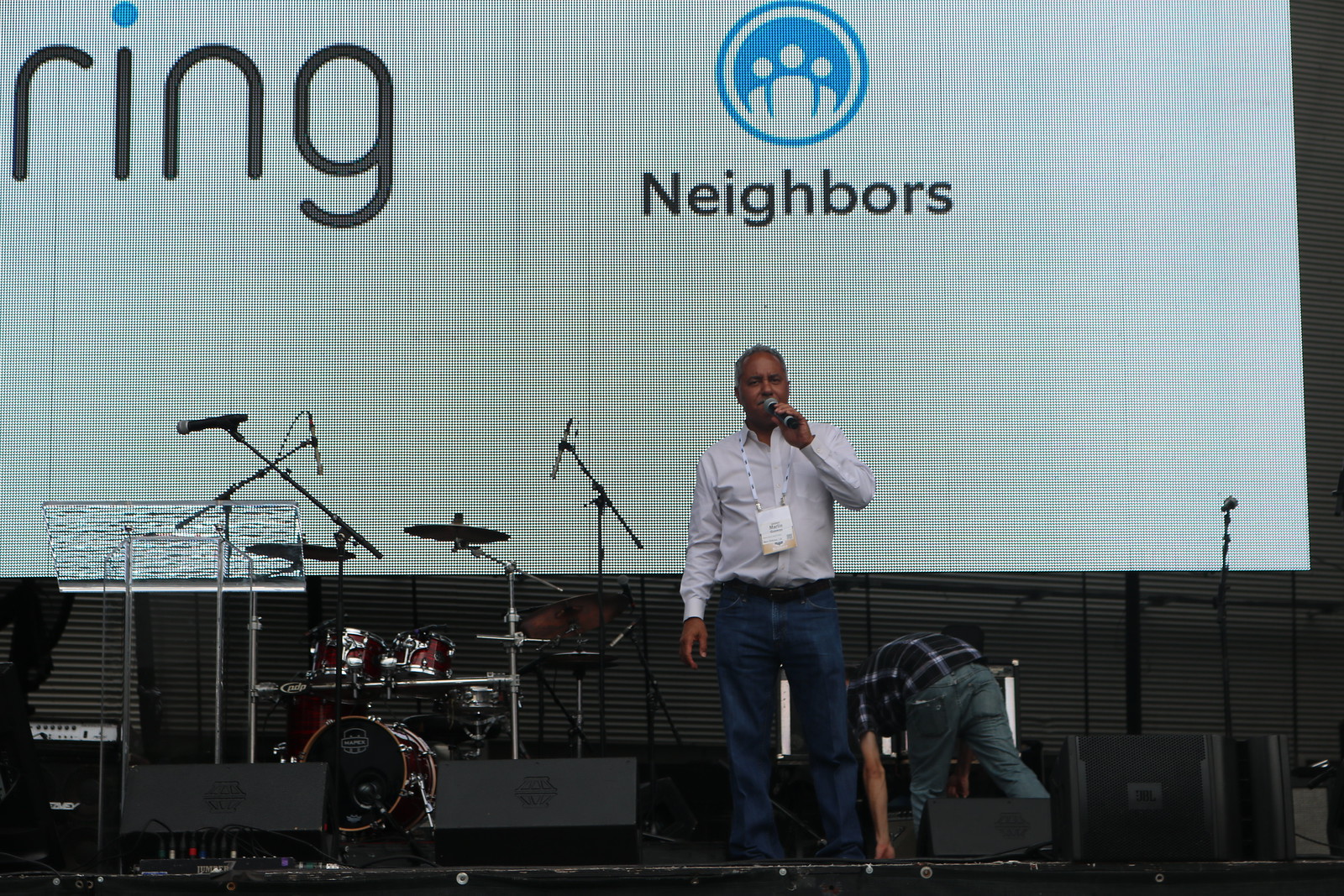The image showcases a dark-skinned man with gray hair standing on a stage, holding a black microphone to his mouth with one hand while the other hand hangs straight down by his hip. He is wearing a white long-sleeve button-up shirt and blue jeans, with a lanyard around his neck that has a white card at the bottom. Next to him on his left is a clear plastic podium and a drum set equipped with microphones pointing towards it. On the right side of the stage, another man wearing a black shirt and blue jeans is bending over, appearing to adjust some musical equipment with both hands on the ground. Behind them is a white backboard featuring the word "Neighbors" in black text, a blue circle with a logo consisting of three circles and four points inside, and over in the upper left corner, the word "ring" with a lowercase 'r' and a blue dot over the 'i'. The scene suggests a conference or festival setting.